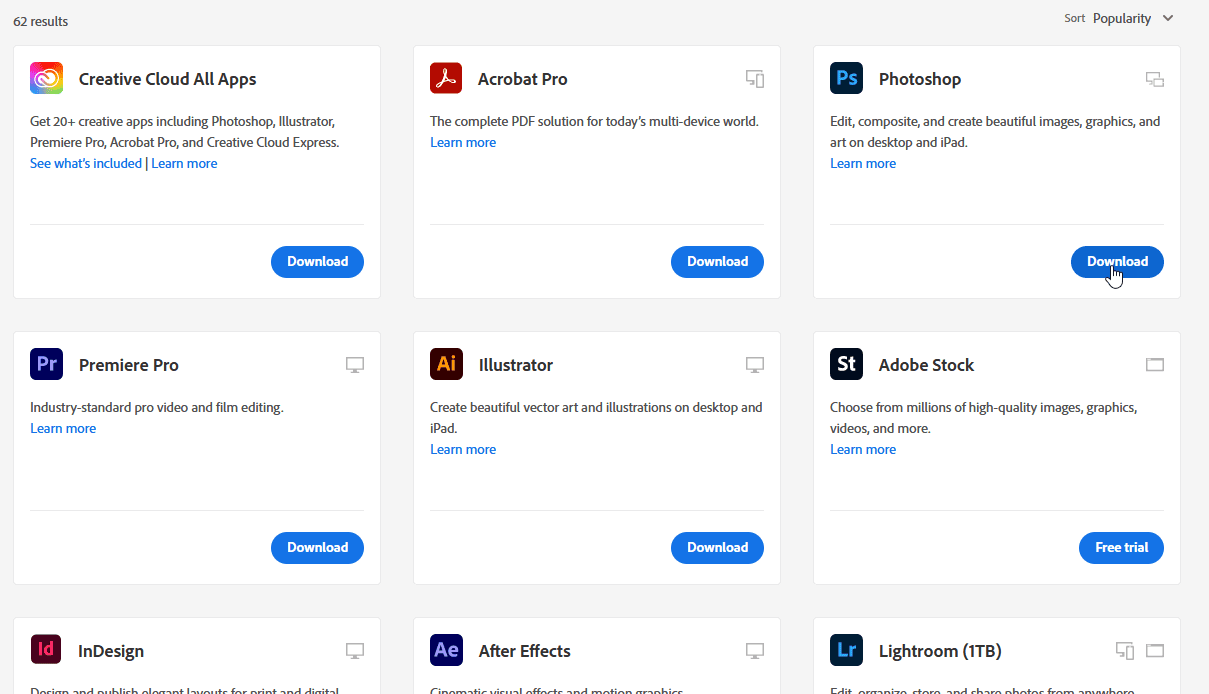In this image, a screenshot of a Google Play Store or similar app store interface is depicted against a white background. At the top in black font, it states "62 Results," and to the far right, there's a "Sort by Popularity" option accompanied by a drop-down arrow. The screenshot displays a grid of six downloadable applications.

The first application listed is "Creative Cloud All Apps" in black font. Following that, "Acrobat Pro," "Photoshop," "Premiere Pro," "Illustrator," and "Adobe Stock" are listed. Each application is positioned within a white background and features a distinctive blue cylindrical "Download" button in the bottom right-hand corner. Specifically, the Photoshop download button has a mouse pointer with a hand icon hovering over it, indicating user interaction.

Additionally, at the bottom section of the screenshot, more applications like "InDesign," "After Effects," and "Lightroom" are available for download. All applications presented are part of the Adobe suite, characterized by their respective download buttons placed consistently in the same location. The overall interface suggests a neatly organized and user-friendly layout, offering easy access to various Adobe software products.